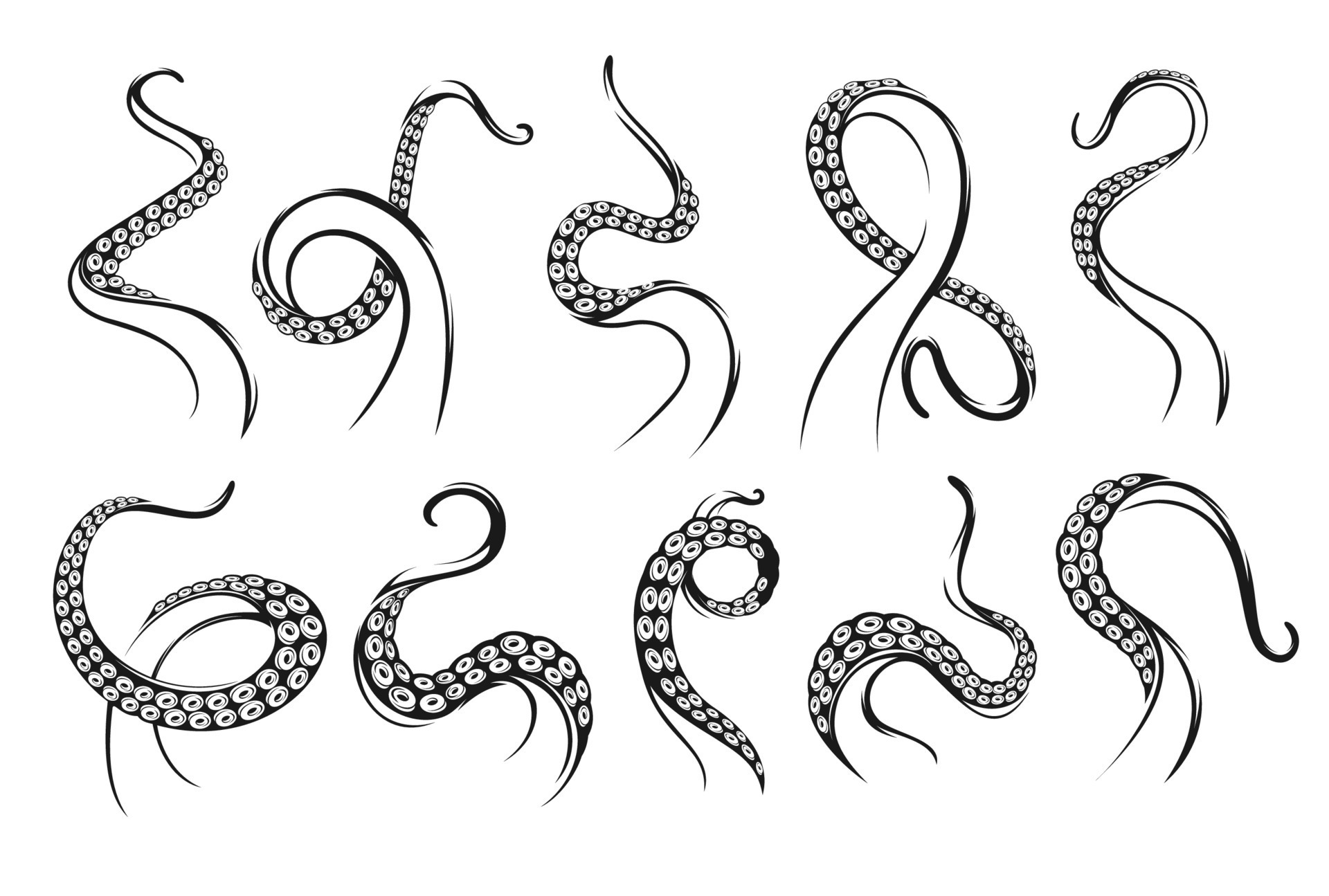The image is an intricately detailed pen and ink (or possibly computer-generated) black-and-white drawing, showcasing ten octopus tentacles arranged meticulously in two rows of five. Each tentacle is uniquely curved and twisted into various shapes, resembling an artistic interpretation of letters and symbols such as S, D, 8, G, E, and V. The tentacles are consistent in size and feature a distinctive pattern of suction cups that resemble tiny circles, adding to their intricate texture. The drawing focuses solely on the tentacles, omitting any depiction of the octopus itself, and is rendered in a precise black ink on a flat white background, emphasizing the contrast and the complexity of the shapes and forms.